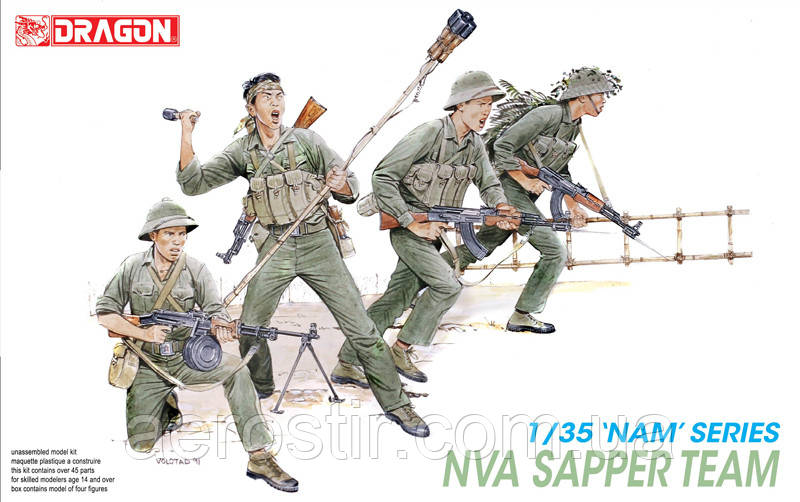The image features a detailed depiction of four Asian soldiers, likely from a model kit, all dressed in olive green uniforms with varying headgear. Three soldiers wear green bucket hats, while the fourth, who is about to throw a grenade from his right hand, sports a bandana. This soldier, also holding a propeller or rocket device in his left hand, keeps his machine gun strapped to his back. The group appears to be advancing towards the right, with each soldier equipped with rifles. One soldier, positioned on the ground and kneeling, wields a machine gun with a drum barrel. Another soldier adorned with camouflage foliage on his helmet and back is seen running forward. The background includes a bamboo ladder on the right and sparse grass and dirt suggestive of a combat zone. In the top left corner, a red rectangle contains the word "dragon" in white letters next to an emblem of a dragon. The bottom left corner, though harder to decipher, mentions "arrowster.com," while the bottom right clarifies the context with "1/35 NVA Sapper Team NAM Series" in various colored text.